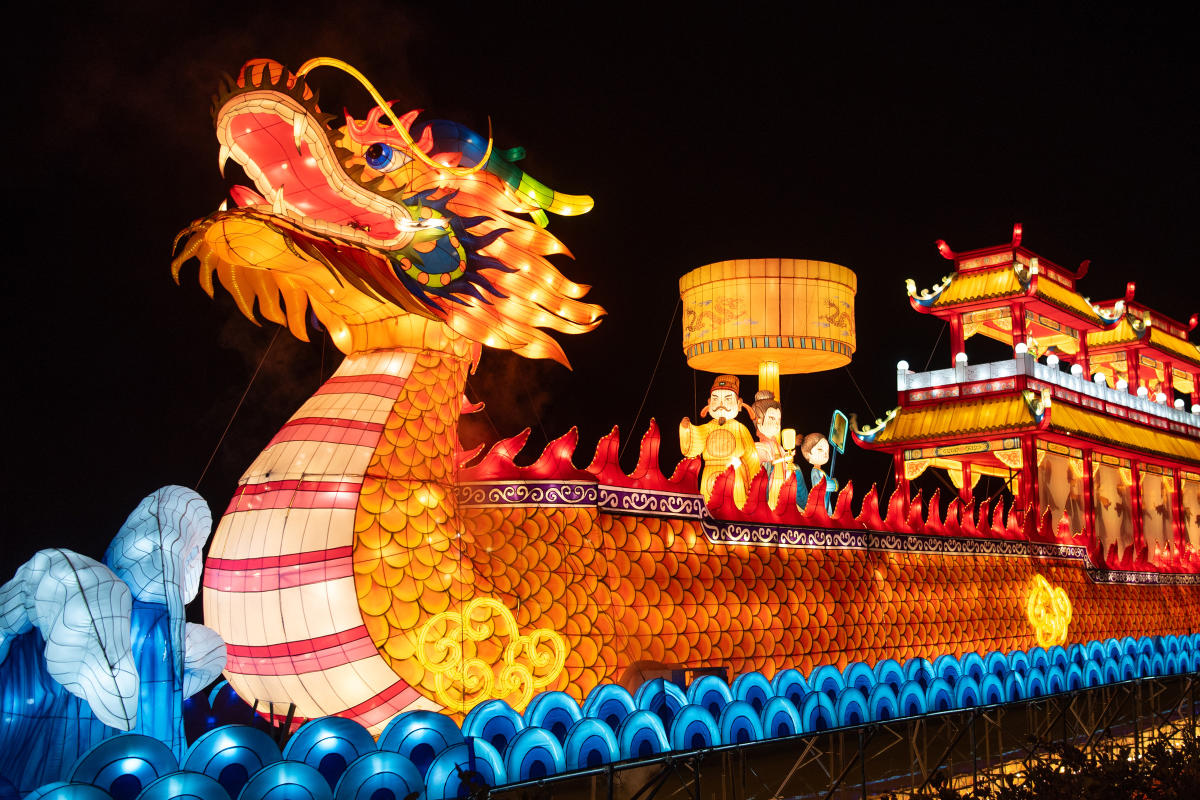A vibrant, large-scale artistic representation of a dragon boat is beautifully illuminated. The bow of the boat features an intricately designed dragon head with its mouth open wide, showcasing sharp teeth and fierce expression. The dragon's eyes are strikingly blue, setting a bewitching gaze. The sculpture boasts a medley of vibrant colors, predominantly yellows and oranges, which simulate the fierce glow of flames emerging from the dragon's mouth and scales. The body of the dragon merges seamlessly into a boat structure, sailing over simulated ocean waves crafted from half-circle forms spread across the base. These wave patterns mimic the movement and appearance of dynamic ocean water. Aboard the dragon boat are figures dressed in traditional Asian attire, evoking the rich cultural heritage and historical asthetics of an older era in Asia. The scene is an extraordinary fusion of art and tradition, capturing the enchanting spirit of dragon boat festivals.